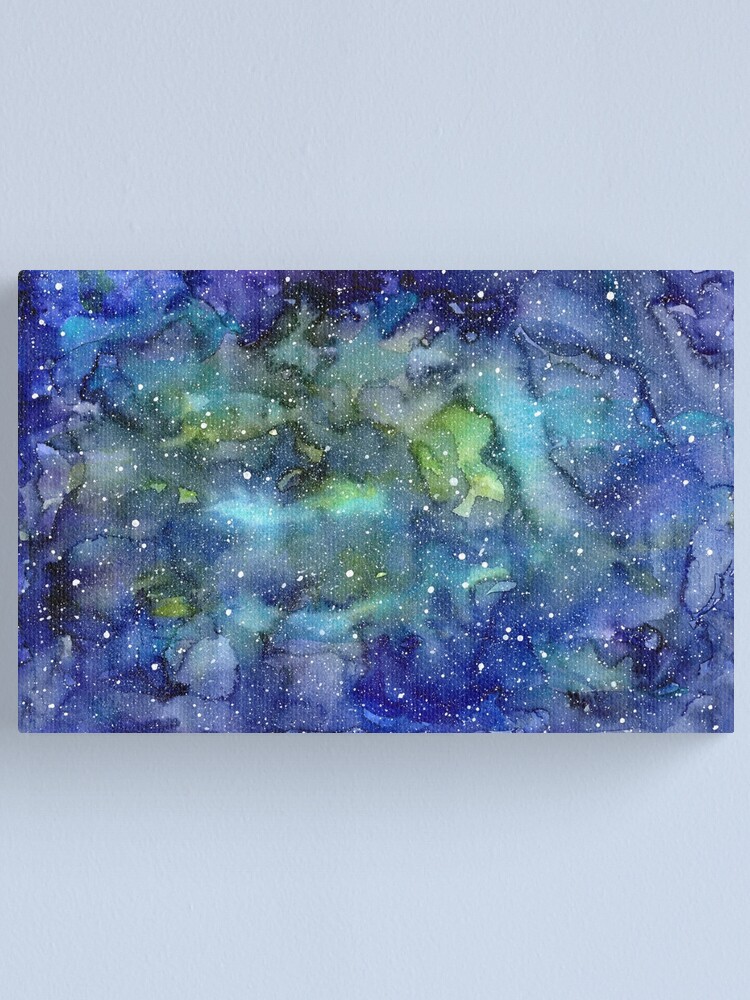The photograph captures a vertically-oriented, textured white canvas mounted on a stark white wall. The canvas features an intricate painting that merges elements of outer space and floral abstraction. This cosmic artwork primarily displays a galaxy or nebula, blending hues of blue and green with accents of light blue and teal. Stars are represented by an array of white dots scattered throughout the composition. The design intriguingly suggests overlapping floral patterns, interspersed with the vibrant colors of flower petals in purple and teal, merged seamlessly with the space theme. This fusion, coupled with sparkles and varied colors, enhances the abstract and ethereal quality of the painting, emphasizing the depiction of a mesmerizing galaxy. The detailed ridges and bumps of the textured canvas add depth and dimension to the celestial portrayal, making it a striking piece of art on an otherwise bare wall.